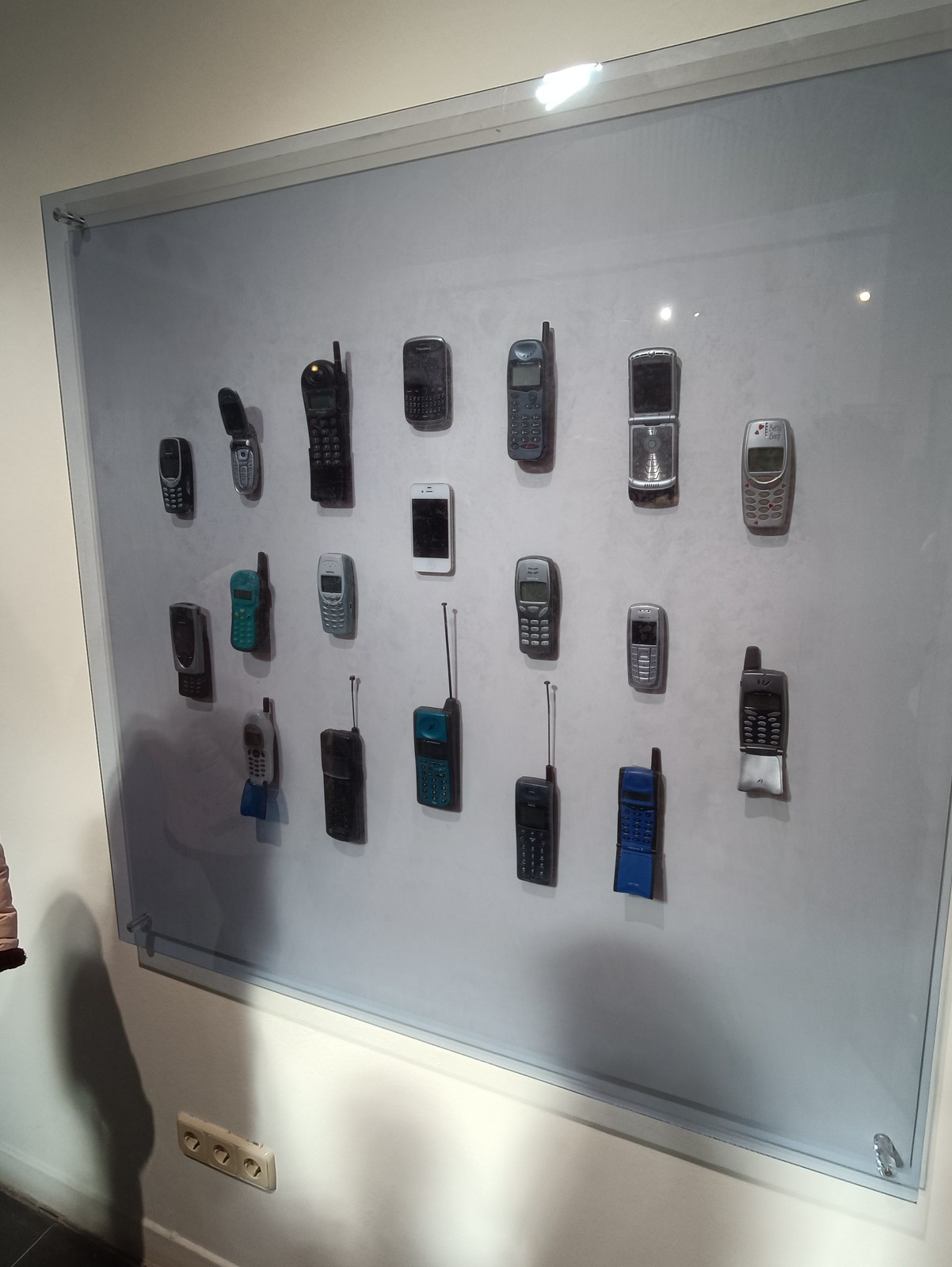The photograph features a detailed display of approximately 20 vintage cell phone models, meticulously arranged on a stark white wall. Encased in a clear, glass-like perspex cover, the collection spans several decades, prominently showcasing iconic devices from the 1990s. The exhibit includes a variety of flip phones, classic Nokia models, and the renowned Motorola RAZR. Additionally, an old BlackBerry and a first-generation iPod can be seen among the assortment. The silver and green hues of the phones contrast with the plain background, and the devices are spaced equidistantly for a neat, organized presentation. Shadows on the wall suggest the presence of onlookers, who add a sense of interaction with the nostalgic display. The photograph is taken from a slight diagonal angle, capturing the depth and careful curation of this vintage mobile phone collection.